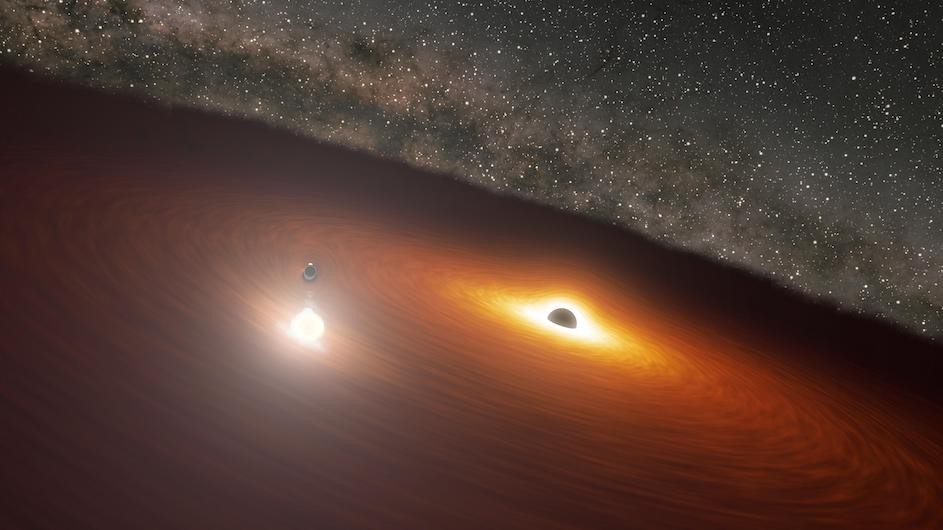This captivating astronomical image appears to capture a scene deep within a galaxy, characterized by a dramatic array of glowing clouds and celestial phenomena. Dominating the lower two-thirds of the image is a swirling disc of incandescent colors—primarily orange, red, and brown—indicative of cosmic matter being drawn into a central, darker area. On the left side of the disc, prominently shining is a bright white-yellow star. Nearby is another intriguing celestial body: a darker, blackish glob which could be interpreted as a black hole, evidenced by the radiation and glowing light encircling it. This suggests the presence of an accretion disc with matter spiraling into the black hole. To the right, a large glowing area with a black center emits a rich orange light, adding to the scene's visual intrigue.

Emerging from one of the swirling arms of the disc is a bright, undefined object—possibly a moon or even a spacecraft. The upper right quadrant of the image serves as a stark contrast to the vibrant chaos below; it resembles a serene night sky dotted with tightly clustered stars. The deep purples and blacks of this region, sprinkled with countless specks of light, suggest that this is either part of the galaxy's arms or possibly the galaxy's core. Overall, the image portrays the dynamic and complex environment of a galaxy's core, with the interplay between stars, black holes, and cosmic matter creating a stunning celestial tapestry.